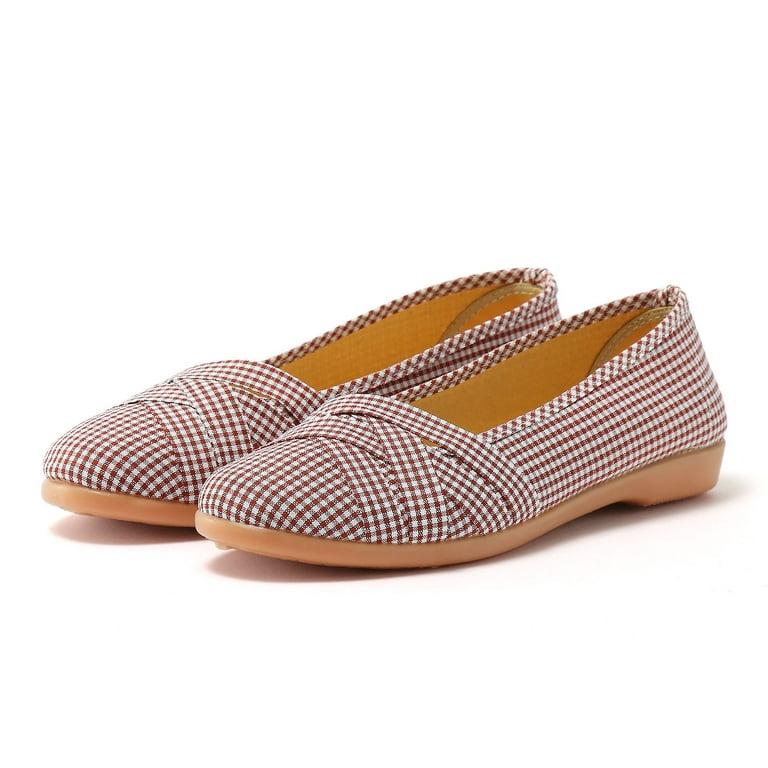This photograph features a pair of women's slip-on clogs with a distinctive red and white checkered pattern on the exterior fabric. The checkers are small, approximately two millimeters each, alternating between red and white. The front of the clogs showcases a crisscross detail with about five overlapping stripes in the checkered pattern. The inside of the clogs appears to be lined with a light brown leather-like material, offering a comfortable fit. 

The soles, slightly heeled, are made of a light peachy pink rubber, providing durability and subtle contrast to the vibrant upper pattern. The shoes are positioned side by side on a solid white background, casting shadows around them, suggesting a minimalist style suitable for a catalog or website presentation. The overall color palette prominently features the red and white checkered design, complemented by the light brown and peachy tones of the sole and interior materials. Subtle details like the meticulous stitching contribute to the quality appearance of the clogs.